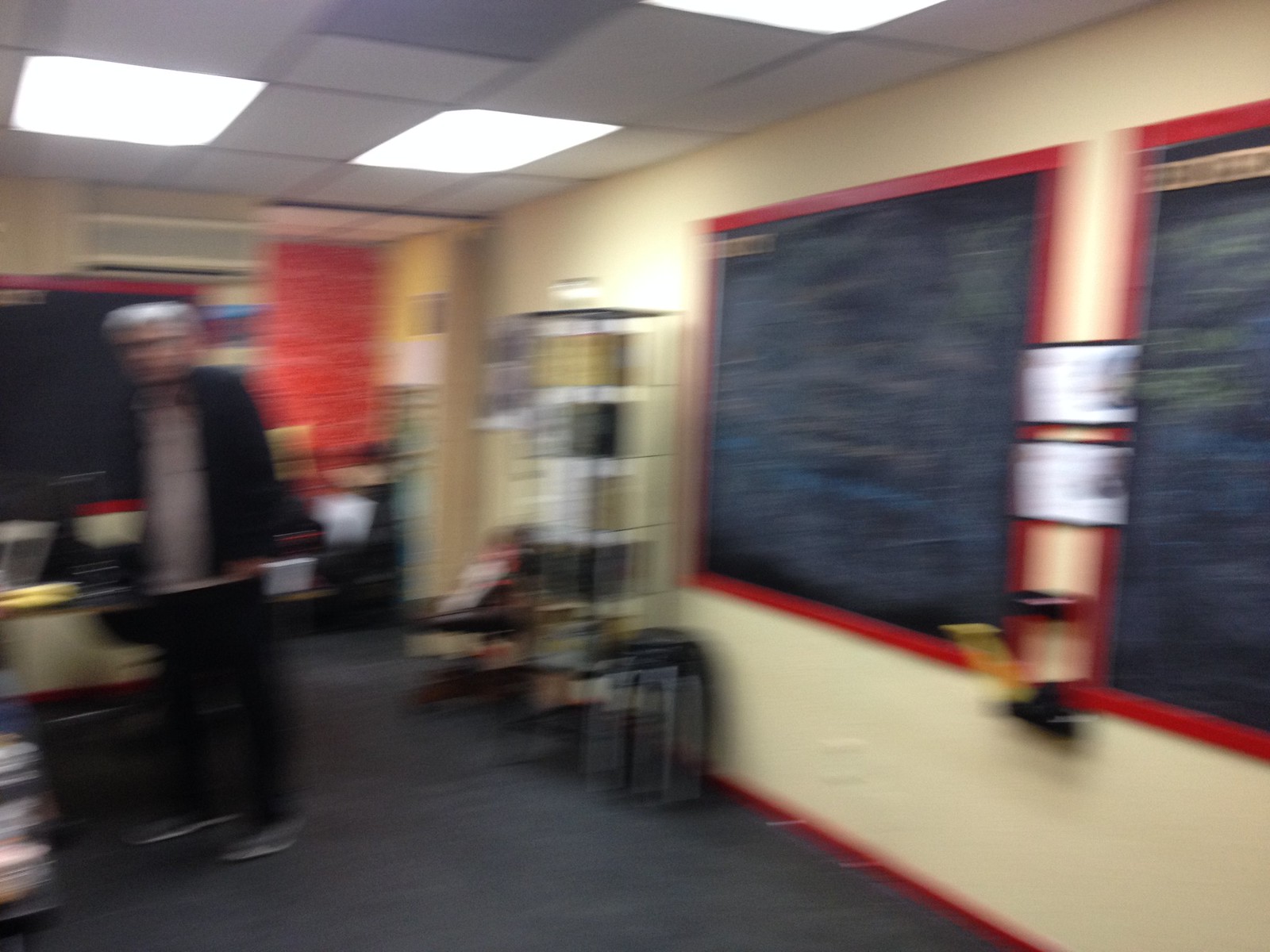The blurry photograph appears to be taken in a classroom or an educational setting. Dominating the right side of the image are two large blackboards with extensive writing, both outlined with a red border. In the middle of these blackboards stands a bookstand, possibly holding books or other materials. To the back left area, there is another blackboard, which may be portable. The ceiling is lit by fluorescent lights, and the floor is covered in gray carpet. An older man with gray hair and glasses is positioned on the left side of the image; he's dressed in a black jacket, light brown or gray shirt, black pants, and gray shoes. Standing behind him, there seems to be storage for books or school supplies, though the exact details are indistinguishable due to the blurriness of the photograph.